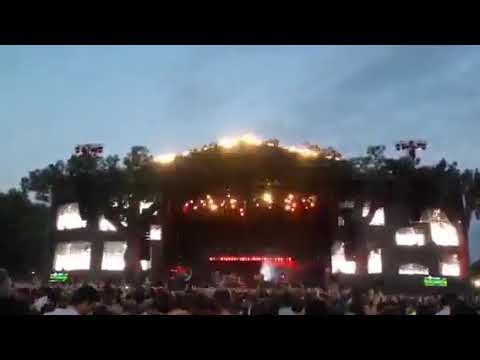The image depicts an outdoor concert at an evening festival, held in a stadium surrounded by a gentle tree line and set against a backdrop of a partly cloudy sky. The focal point is a brightly lit stage situated in the middle, emanating a vibrant array of red, yellow, and orange lights, casting an inviting festival atmosphere. The stage, bustling with activity, is complemented by several brightly lit monitors on either side—approximately eight on the right and six on the left—enhancing the visual experience for the large crowd below. Audience members, visible from behind, are captivated by the performance unfolding on stage. The stadium's expansive setup merges with the softly illuminated evening, indicating the event is taking place at dusk, just as the day transitions into night.